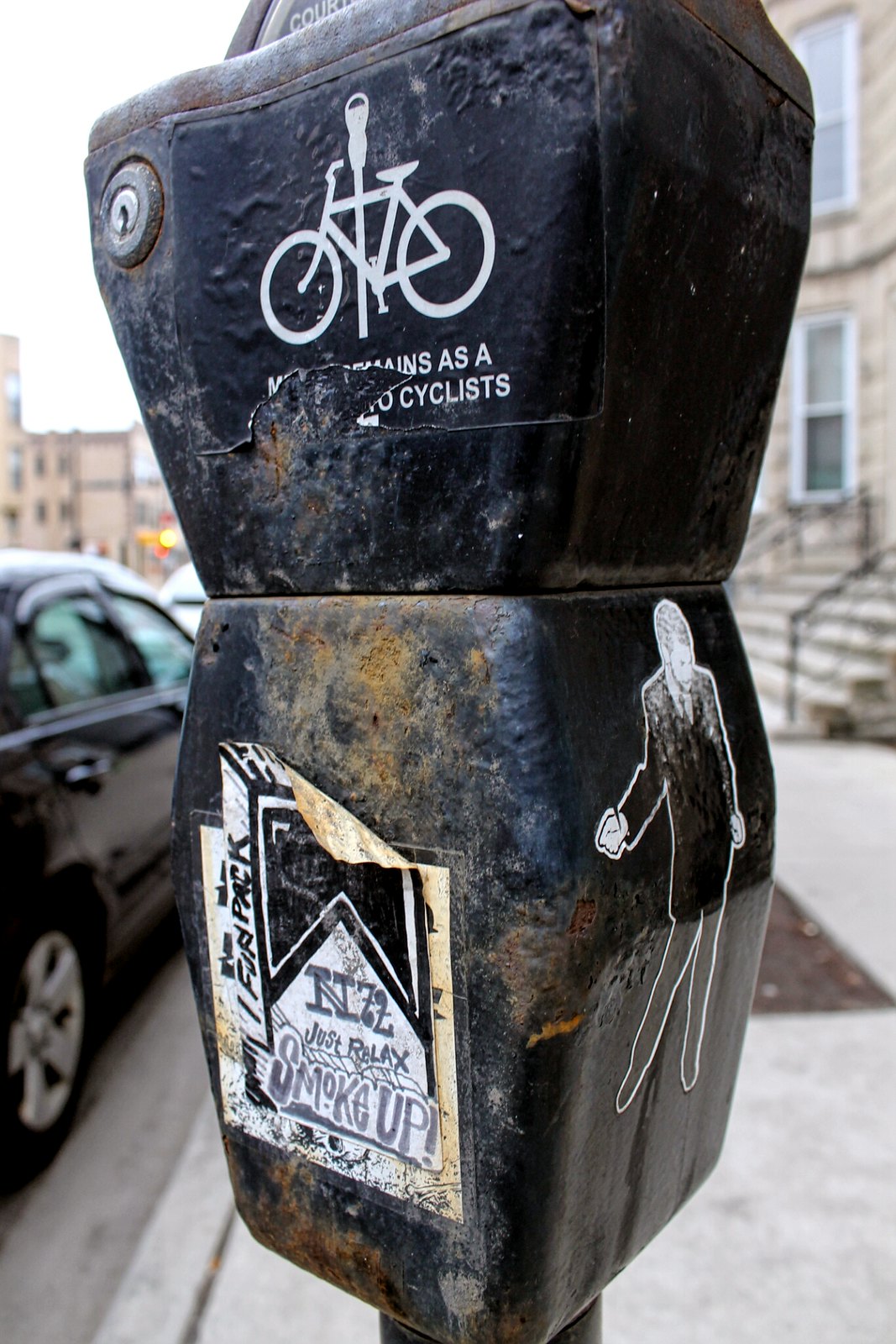The image features a prominently aged black parking meter positioned centrally. The meter shows signs of rust and wear, indicating its old age. Adorned with several stickers, the top section bears a black sticker with an illustration of a bicycle and a parking meter in white, suggesting a connection to cyclists, though partially torn and obscure in meaning. The right side of this section includes a keyhole. Below, on the thinner side, a sticker portrays a man in a black suit, his identity unclear, possibly a performer or a dancer. The bottom of the meter displays a poorly peeled sticker with a black ribbon design that has handwritten messages, "One Fun Pack" and "Just Relax, Smoke Up," likely referencing marijuana. The entire scene is framed by the sidewalk, a parked black car, and buildings in the background, harmonizing with the urban setting.